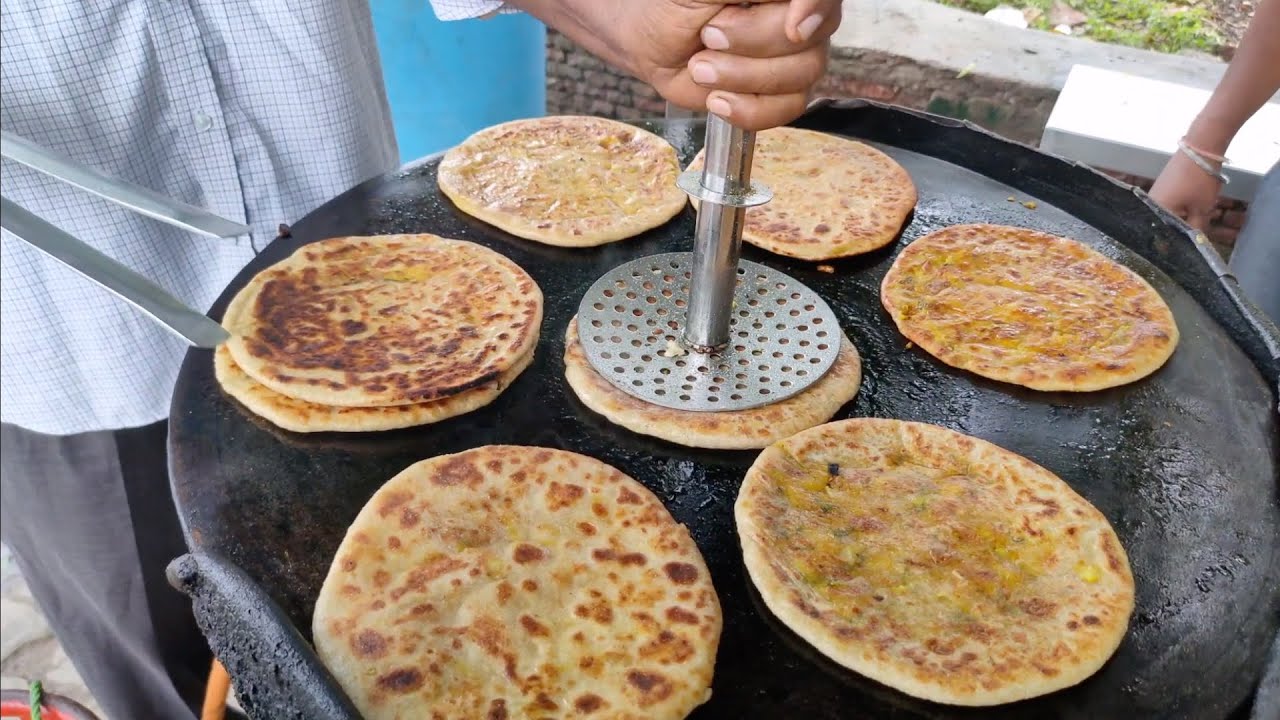In the image, a man dressed in a checkered light blue shirt and gray slacks is cooking flatbread on an outdoor black griddle. The griddle, aged and heavily used, holds about eight to nine pieces of flatbread in various stages of browning. The man is pressing one of the central pieces of flatbread with a silver, perforated stainless steel press in his left hand while holding tongs in his right hand. Only part of his left side is visible. To the right, partially visible is a woman's arm adorned with a silver and gold bracelet, likely indicating her presence in the scene. Surrounding the cooking area, there is a half brick wall topped with a white surface, suggesting a patio setting. Additionally, there is a green string in the bottom left corner, adding a minor detail to the outdoor scene. The flatbreads appear to be brown and evenly cooked on a flat skillet pan, indicating they are nearly ready to be served as part of a potential street food setup.